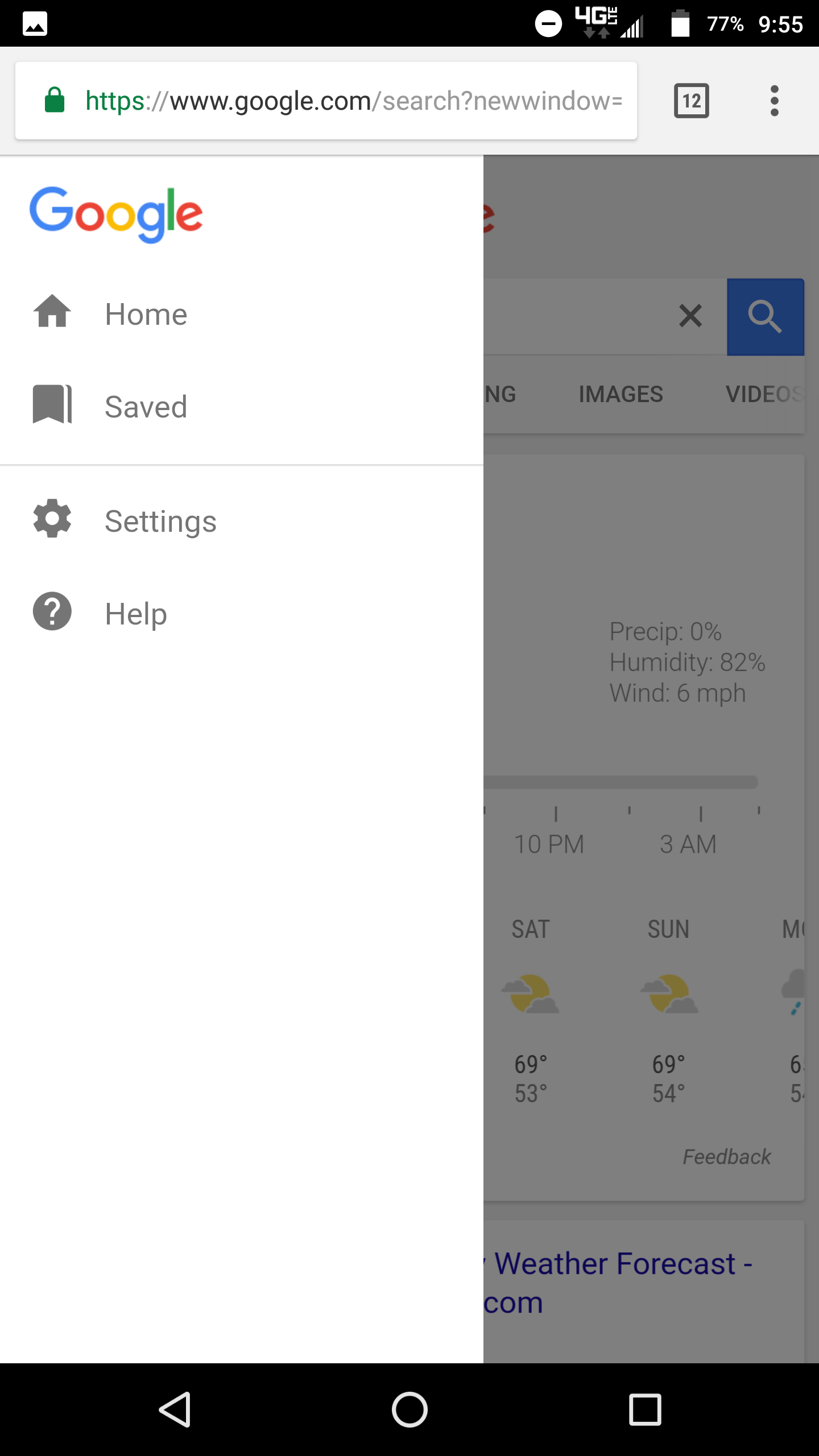The image depicts a screenshot of a mobile device. At the top, there is a black header featuring an icon for images or photos. On the right side of this header, the device's battery level is displayed at 77%, the current time is 9:55, and the 4G network indicator is visible. Below the header, there is an address bar reading "www.google.com/search" in white text. To the right of the address bar, there is a small black box with the number 12 in a white background, followed by three vertical dots.

On the left side of the screen, the colorful Google logo is present, designed with blue, red, yellow, and green. Beneath this logo, there are menu options listed as Home, Saved, Settings, and Help. In the background, part of a webpage is visible, displaying weather information. The weather forecast indicates 82% humidity and wind speeds of 6 miles per hour. For Saturday, the weather is partly cloudy with a high of 69°F and a low of 53°F. For Sunday, it is also partly cloudy with a high of 69°F and a low of 54°F.